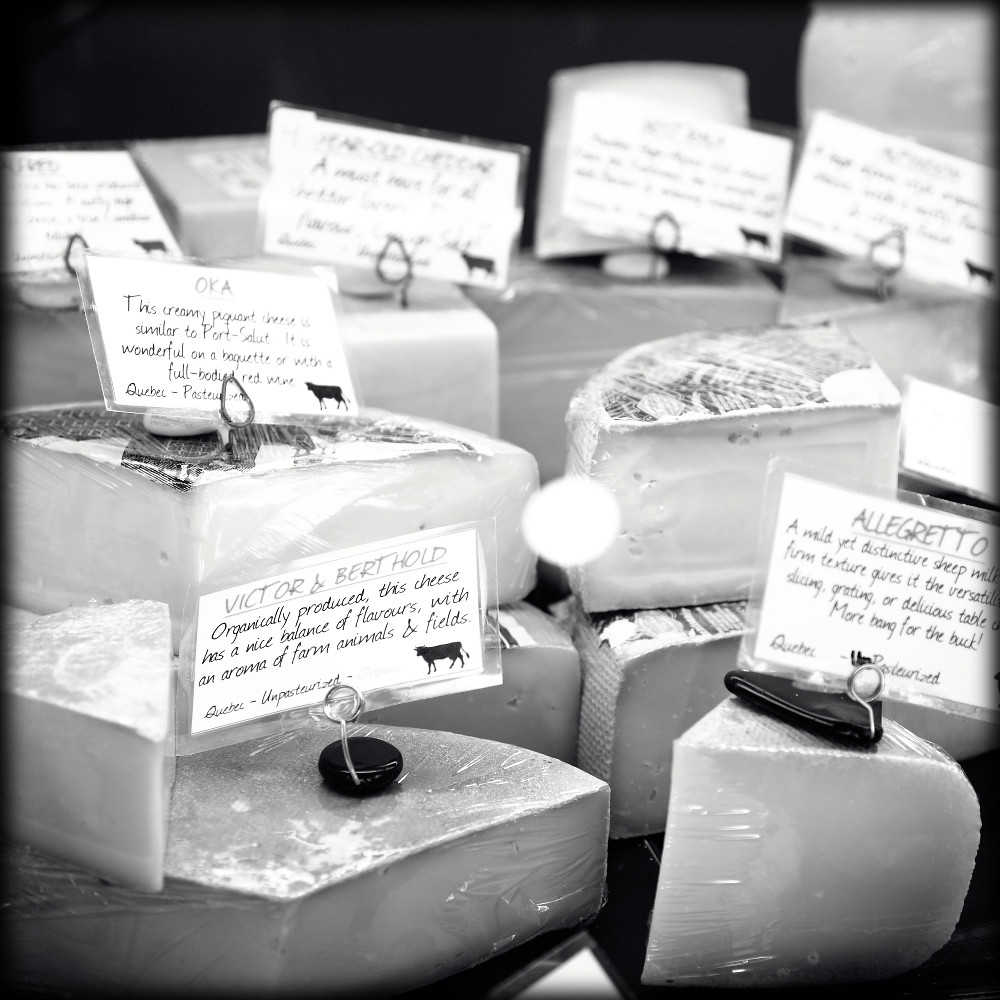The photograph showcases a detailed display of various cheeses, artfully arranged on a shop table. Each cheese, presented in its original wheel form, has been cut into quarters, chunks, or slices, and is wrapped in cellophane. Small black stones with metal rings are placed on top of each piece, holding laminated white cards that provide information about the cheeses. Each card, featuring a black silhouette of a cow in the lower right-hand corner, offers descriptions of the cheese varieties. Notable examples include "Allegretto," described as a mild yet distinctive sheep milk cheese with versatile uses for skiing, grating, or as a table cheese, and "Victor and Berthold," an organically produced cheese with a balanced flavor profile and an aroma reminiscent of farm animals and fields. The image is rendered in black and white, contributing to the rustic charm of this meticulously arranged cheese display.